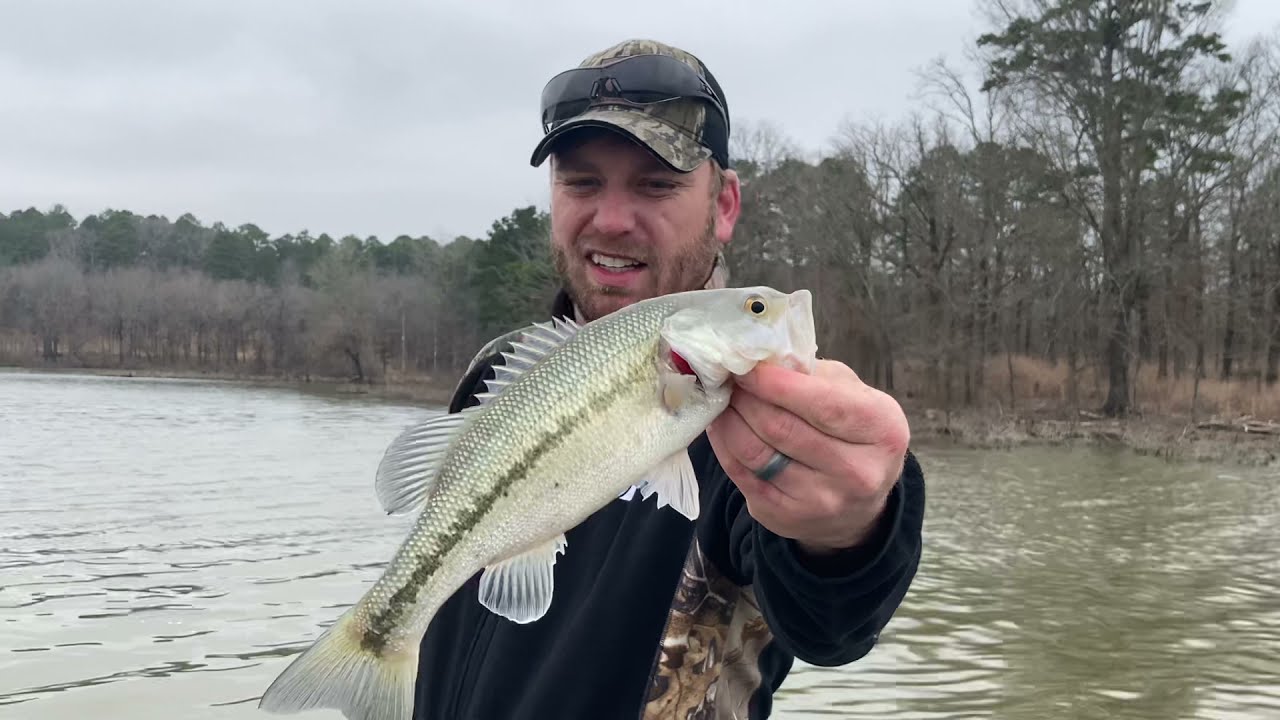In this outdoor scene, a man proudly displays his catch, holding a light-colored fish by the gills directly toward the camera. He wears a camouflage baseball cap adorned with sunglasses, a black jacket with a brown hunting pattern on the sides, and a silver wedding band on his hand. His bearded face sports a look of triumph as he gazes at the fish. Behind him lies a serene, brownish river bordered by a shoreline and flanked by a mix of leafless brown trees and a dense row of green trees. These trees, growing taller toward the right side of the image, stand out against the overcast, gray sky, which adds a moody backdrop to the picturesque scene. Notably, a particularly tall tree rises on the upper right bank of the river, contributing to the depth of the background.